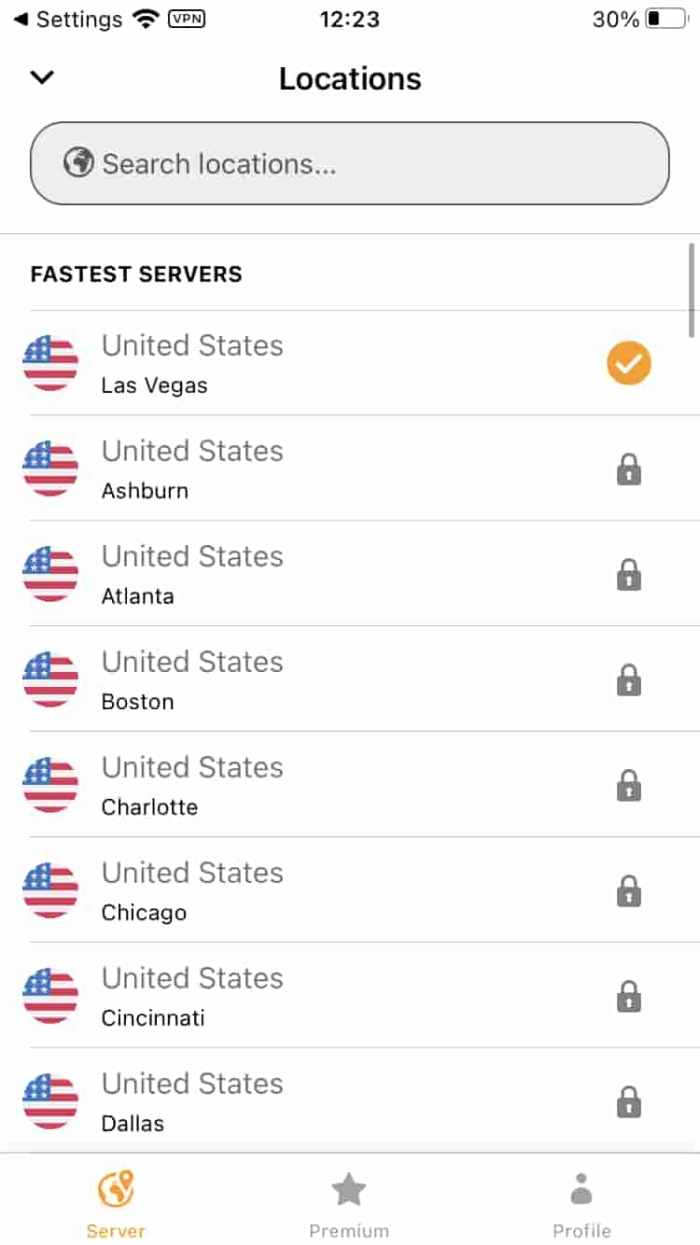This screenshot captures a settings page on a cell phone, specifically focusing on the "Locations" section. The entire interface is set against a white background. 

**Header:**
- At the top left:
  - A black left-pointing arrow
  - The word "Settings"
  - A Wi-Fi symbol composed of radiating rounded bars
  - A black rectangular outline with "VPN" inscribed inside it

- Centered at the top:
  - The time reads "12:23"

- At the top right:
  - "30%" indicating the battery percentage
  - A low-capacity battery icon

**Main Section:**
- Beneath the header:
  - The section title "Locations"
  - Below this, a gray pill-shaped search bar with an earth icon inside, designed for searching locations

**Content:**
- A list titled "Fast Servers," featuring eight locations within the United States. Each location is associated with a circle featuring part of the U.S. flag, showing a segment of the blue field with white stars and red and white stripes.

- The locations listed are:
  1. Las Vegas (selected, marked by a mustard-colored circle with a white check mark)
  2. Ashburn (locked, indicated by a gray lock icon on the right)
  3. Atlanta (locked)
  4. Boston (locked)
  5. Charlotte (locked)
  6. Chicago (locked)
  7. Cincinnati (locked)
  8. Dallas (locked)

**Footer:**
- At the bottom left:
  - A label "Server"
  - An icon of a round circle with a location marker inside

- Center:
  - A star icon labeled "Premium"

- At the bottom right:
  - An icon of a gray figure representing a profile, depicting only the head, torso, and shoulders

This well-organized layout provides easy navigation for selecting and managing VPN locations within the United States.